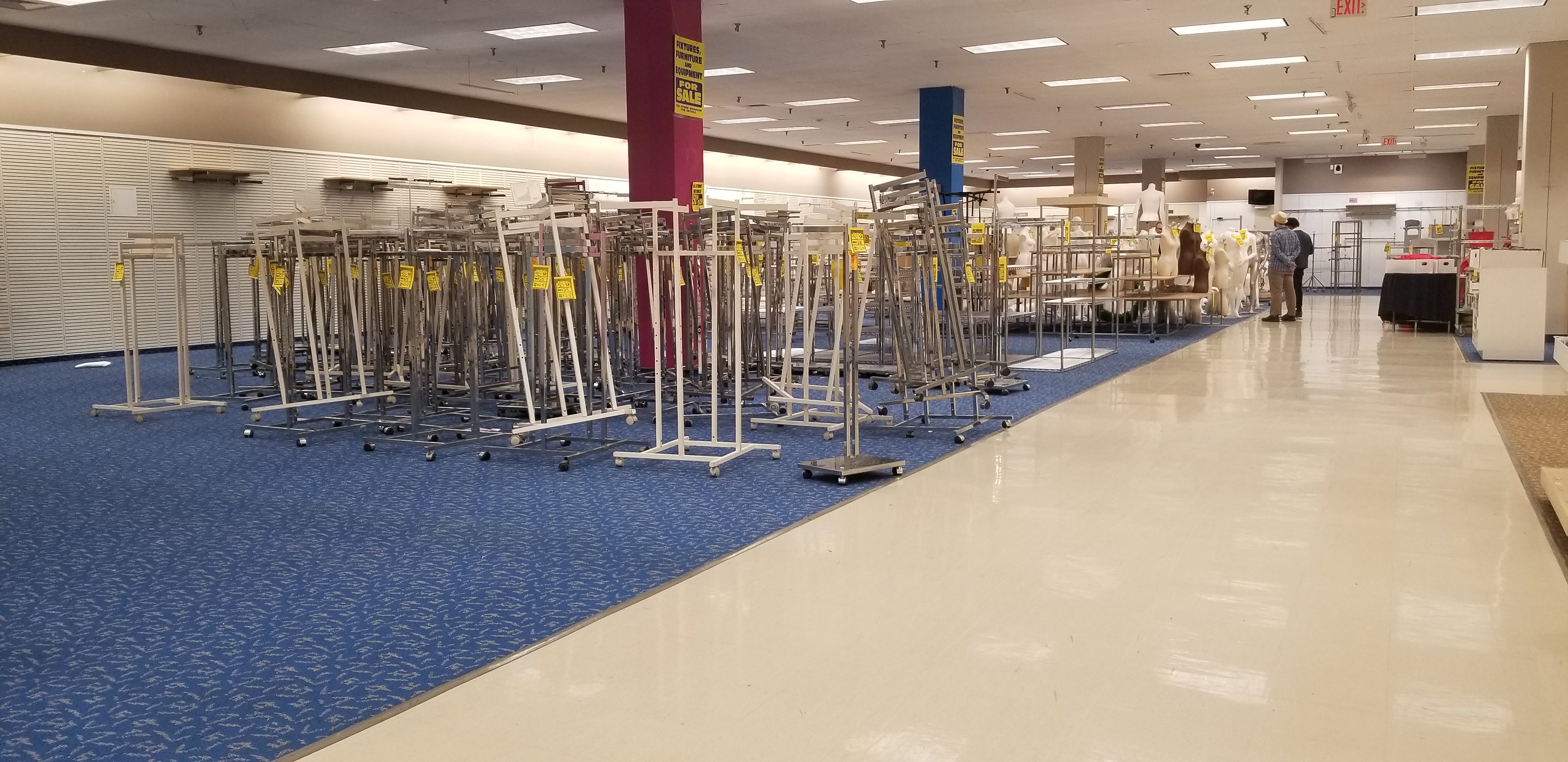The image depicts the interior of what appears to be a large department store. The main focus is a series of tall, wheeled clothing racks with square bases and metal poles, presumably used for displaying clothes. These racks are all currently empty and are tightly arranged in close proximity to one another. The floor beneath them is carpeted, contrasting with a tiled area visible to the right side of the image. In the background, two men are seen conversing and pointing towards the racks, suggesting they might be assessing or organizing the scene. Given the emptiness of the displays and the men's actions, it is possible that the store is either preparing for a major change, such as refurbishment or possibly going out of business. The orderly arrangement and the context provided by the varied flooring indicate a structured retail environment.